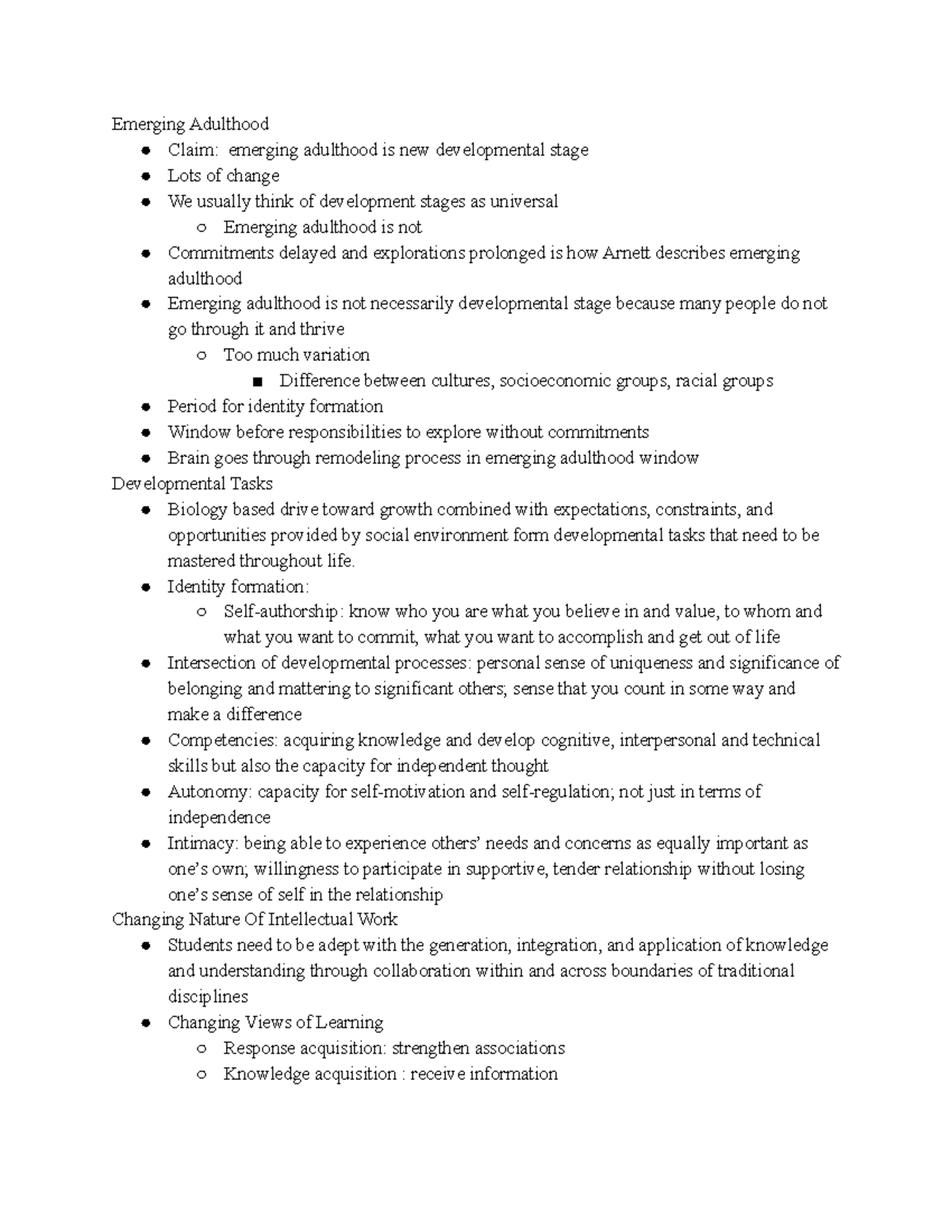Emerging Adulthood: A Detailed Exploration

The text on the white background, with black text and bullet points, elaborates on the concept of emerging adulthood, a relatively new developmental stage characterized by significant changes. Unlike traditional developmental stages considered universal, emerging adulthood varies greatly among individuals. This stage is marked by delayed commitments and prolonged exploration.

Emerging adulthood is not universally experienced; its applicability varies with many individuals not undergoing this stage at all, highlighting the diversity in personal development. The text emphasizes the differences that arise between cultures, socio-economic groups, and racial groups.

This period is seen as a crucial phase for identity formation, providing a window of opportunity to explore without the burden of responsibilities. During this time, the brain undergoes significant remodeling.

Emerging adulthood is shaped by developmental tasks which combine biologically driven growth with the expectations, constraints, and opportunities of social environments. Key tasks to be mastered include identity formation and self-authorship, involving understanding who you are, what you believe in and value, whom you want to commit to, and what you want to accomplish in life.

The intersection of developmental processes during this stage fosters a personal sense of uniqueness and the significance of belonging and mattering to others. A sense of making a difference is crucial.

Competencies developed during this time include acquiring knowledge and skills—cognitive, interpersonal, and technical. Furthermore, the capacity for independent thought, autonomy, self-motivation, and self-regulation are highlighted. This is not solely about independence but also about intimacy—understanding and valuing others' needs and concerns as much as one's own. There's an emphasis on the willingness to engage in supportive, tender relationships without losing one's sense of self.

The text underscores that emerging adulthood is a critical period for personal growth and development, marked by complex intersections of personal and social development processes.